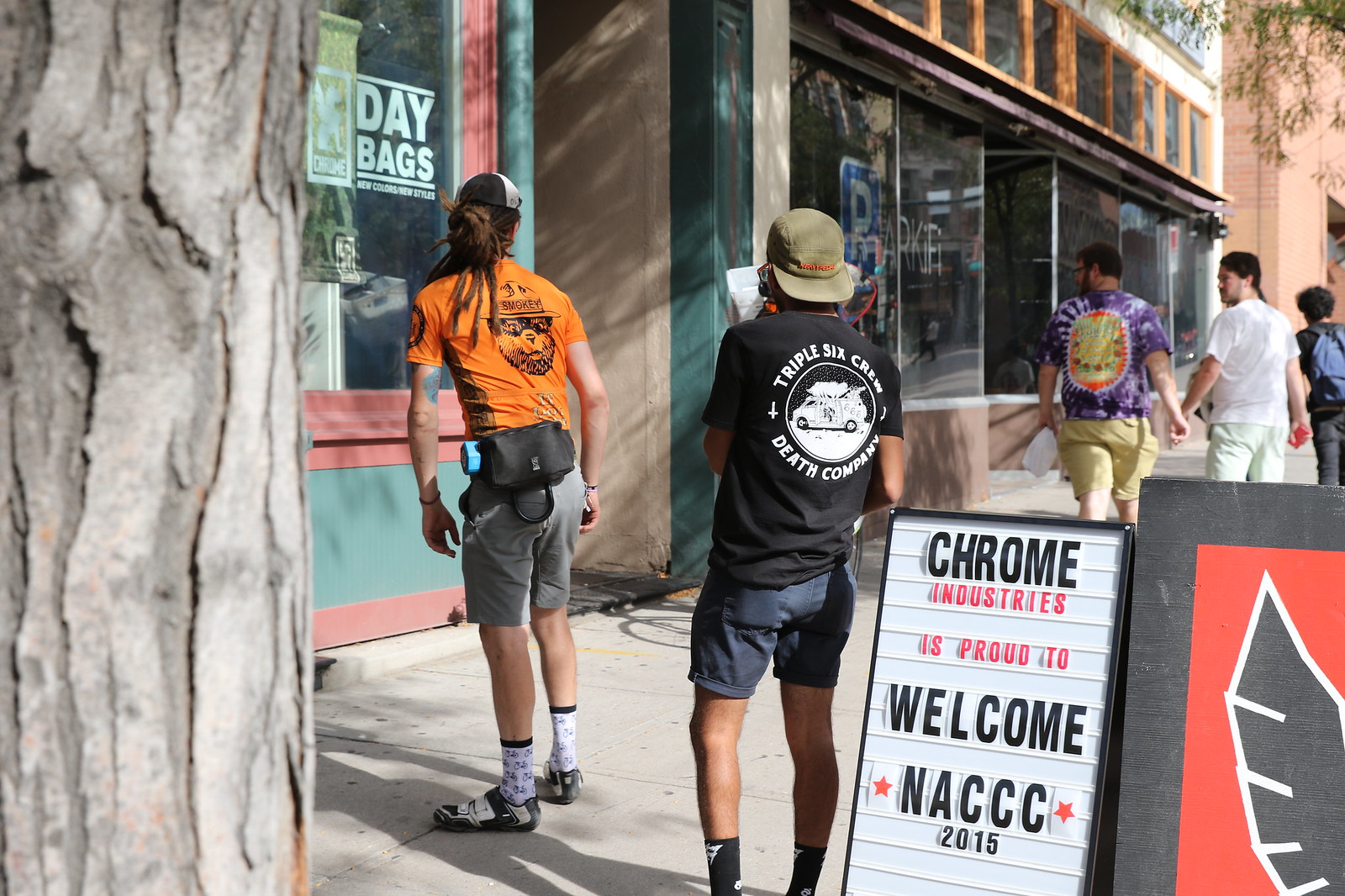The photograph captures a bustling sidewalk scene along a string of shopping centers and outlets on a busy city street. On the left side of the image, a large tree trunk partially obscures the view, creating a natural frame. Prominently in the foreground, two men are standing; one in an orange shirt with a fanny pack, positioned in front of another man wearing a black shirt and blue shorts. Behind them stands a white sign with black and red lettering that reads, "Chrome Industries is proud to welcome NACCC 2015." Adjacent to this, another sign with a partially visible logo can be seen. Further down the sidewalk, a small group of pedestrians is visible, including two men holding hands—one in a white shirt and the other in a purple shirt—and a younger individual with a backpack, likely a teenager or a student. The scene is vibrant with activity, capturing both immediate interactions and distant movements of various people.